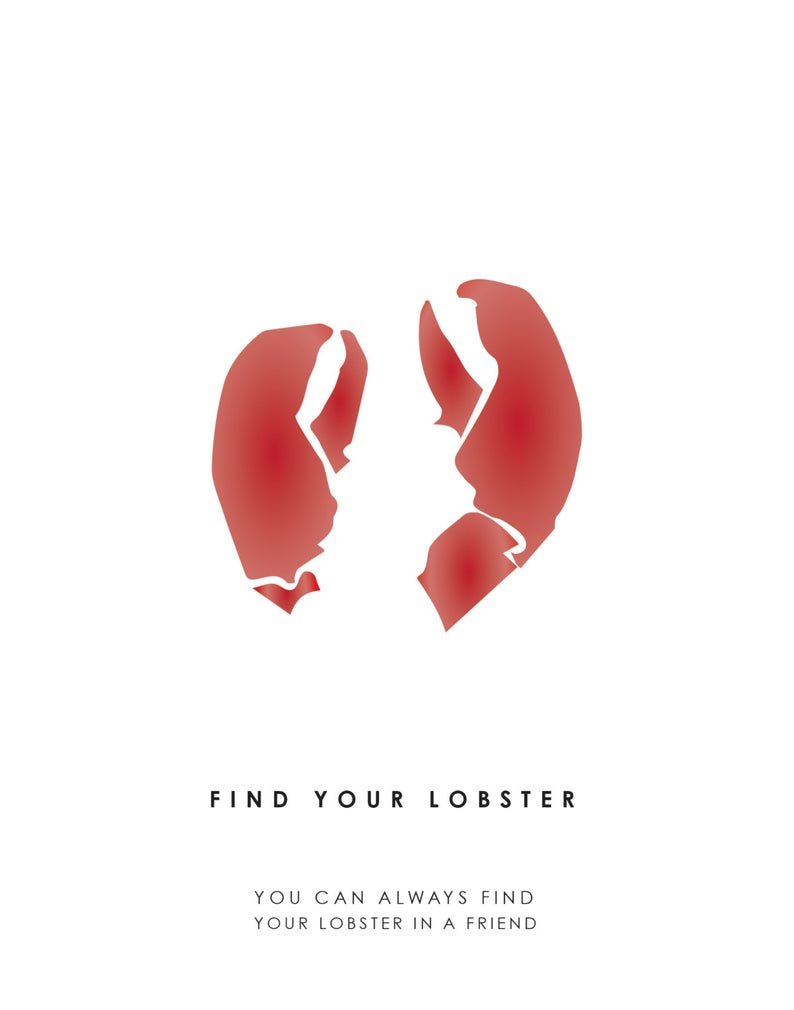The image features a white background with a prominent pair of red lobster claws, positioned to resemble a heart shape. The claws are distinct, with the right one slightly larger, suggesting different functions, such as grabbing and splitting. Below the claws, there is black text in all caps that reads "FIND YOUR LOBSTER." Even further below, in a smaller font, is additional text that states, "You can always find your lobster and a friend." The overall composition of the image appears to promote the idea of finding companionship, likening it to a lobster’s claw, perhaps for an adoption or recruitment campaign. The simplicity and clarity of the design emphasize its message effectively.